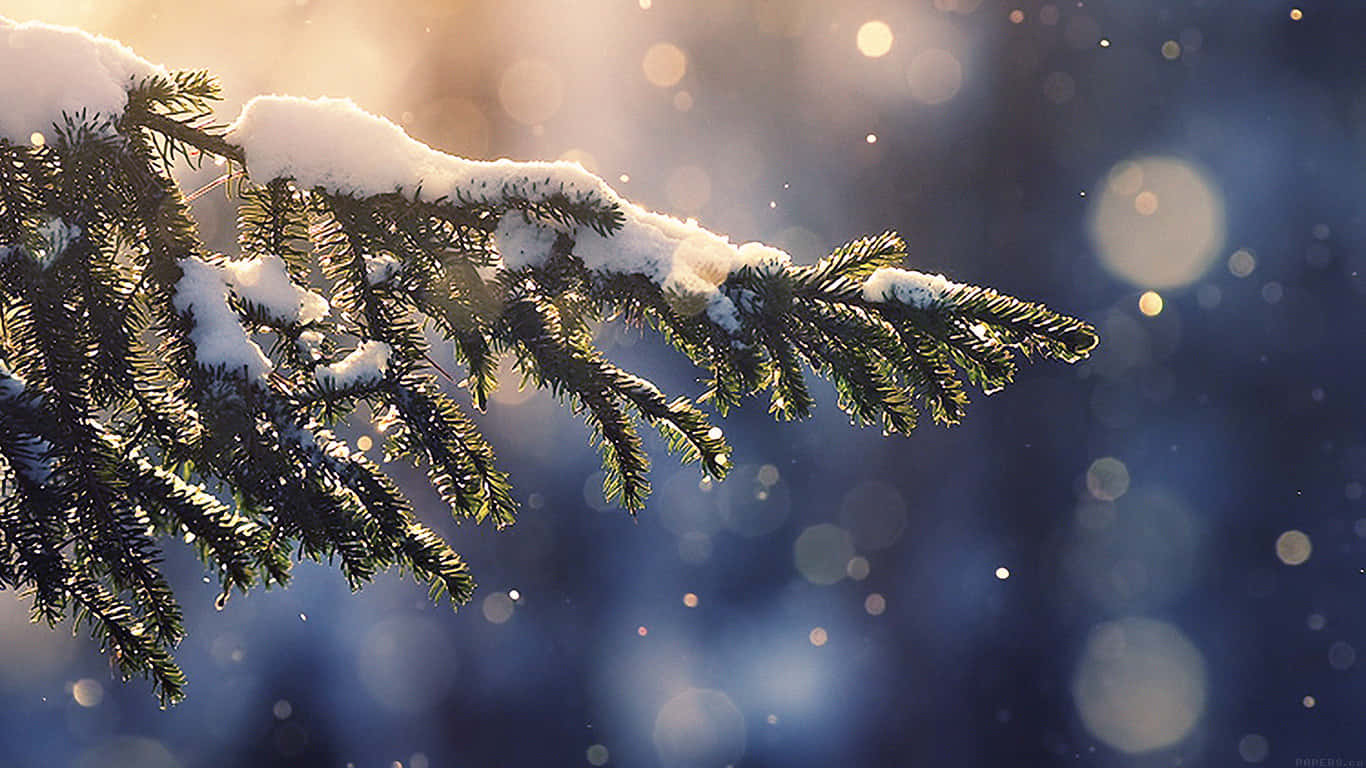This photograph captures a pristine winter scene featuring a snow-covered evergreen branch, reminiscent of a Christmas tree. The branch extends from the upper left and slopes downward toward the lower right, dominating three-fourths of the image. Its lush green needles are adorned with a thick layer of snow, especially prominent on the topmost branch with more scattered across the smaller branches below. The backdrop is a dark blue, blurred to emphasize the branch and dotted with various light flares and speckles that evoke a wintry atmosphere. The white and grayish light spots in the background give the impression of gently falling snow illuminated by ambient light, enhancing the festive and serene mood of the scene.